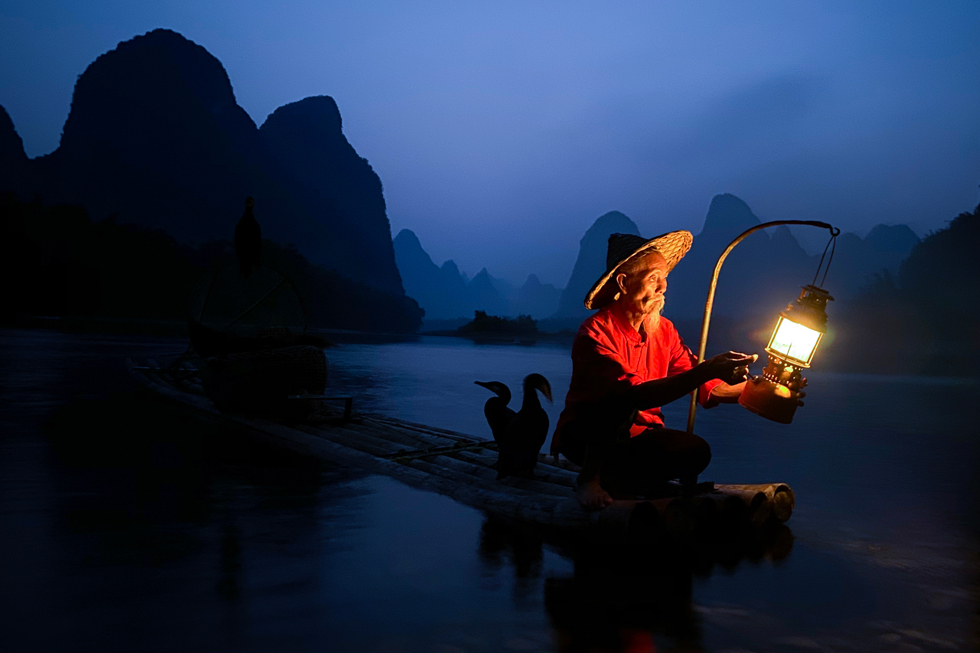In the dim light of night or early morning, an older Asian man, possibly in his 60s or 70s, is crouched on a modest raft made of logs tied together. His attire includes a wide-brimmed, pointy straw hat and a red shirt paired with dark pants. He is tending to an old-fashioned lantern that hangs from a curved wooden rod at the front of the raft, illuminating his face and surroundings. The scene exudes a sense of solitude and serenity, set against a backdrop of still, dark water surrounded by jagged, fog-enshrouded mountains. The atmosphere is heavy with a sense of seclusion; no signs of civilization are visible. Behind the man, three birds with long necks—possibly cormorants—sit quietly, their silhouettes adding to the mystique of the scene. To the left of the man, a small basket is nestled on the raft, potentially holding his belongings. The entire tableau is framed by a dark, foggy sky that obscures the distant mountains and creates an eerie, yet tranquil, ambiance.